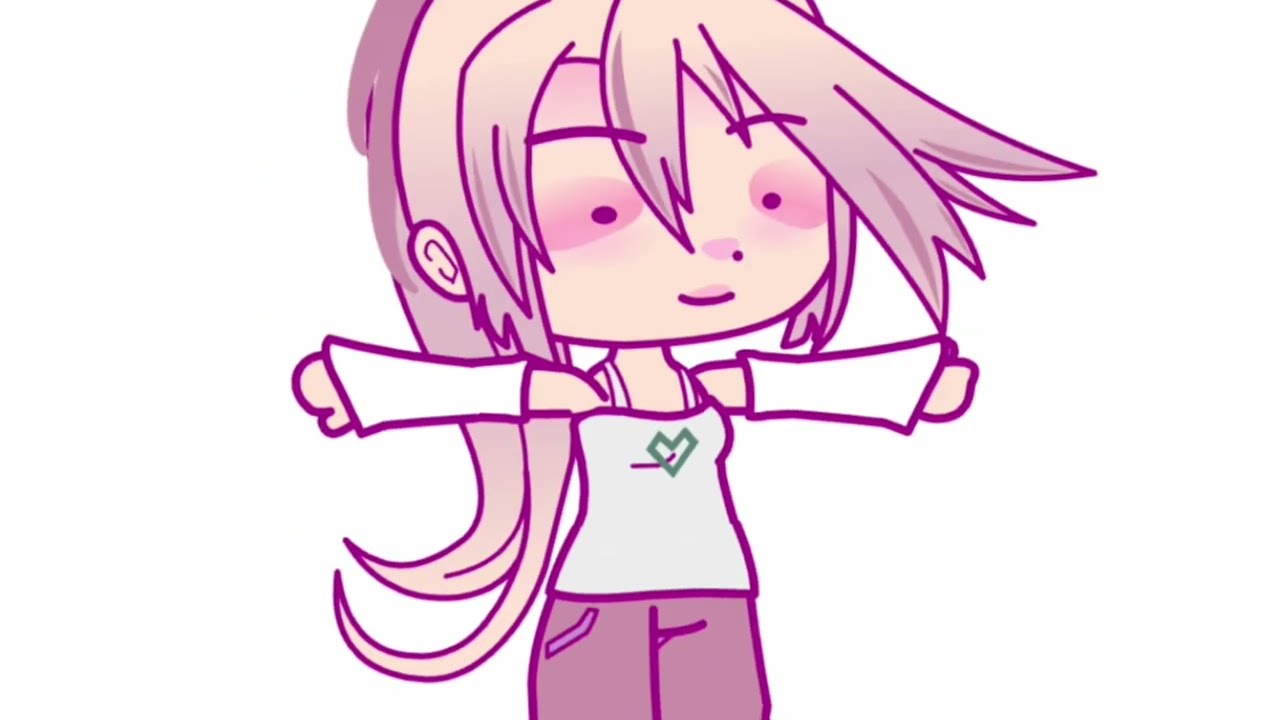This is a digital drawing of a cartoon female character with distinct anime-like features. Her segmented, light purple hair is styled with spiky front bangs and longer curls at the back. She has an oversized head in proportion to her minimalistic body, exhibiting a unique design with black dot eyes and a simple dot for a nose against a pink-shaded face. She wears a seafoam green tank top with a prominent green heart on the front. Her arms are extended to the sides in a T-pose, adorned with white arm warmers that stretch from her wrists to her shoulders, leaving her shoulders bare. She is dressed in purple pants and is set against a white background, invoking a playful, cartoonish vibe.